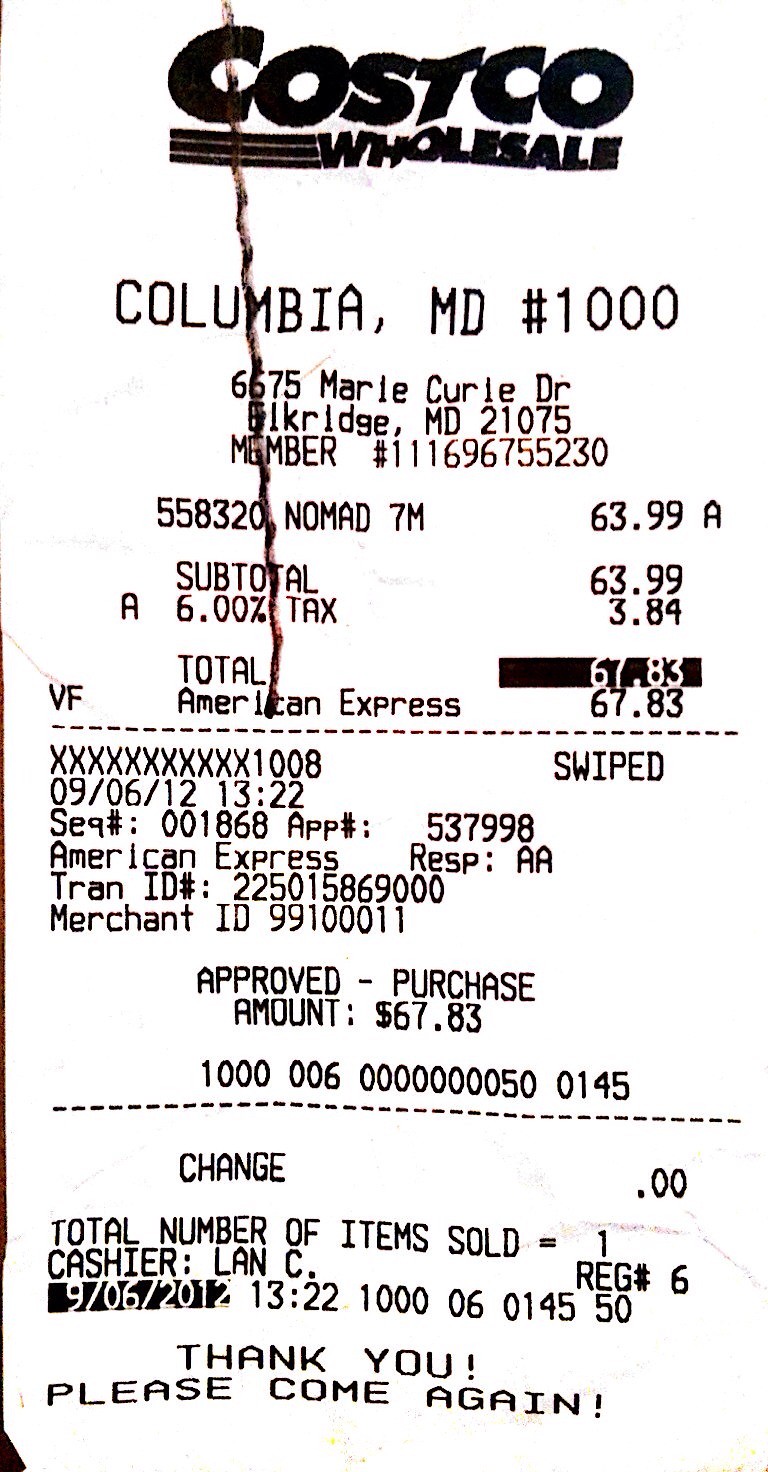This is a photograph of a meticulously scanned receipt from a Costco Wholesale store, ensuring a perfectly clear, artifact-free image with pristine lighting. At the top, the receipt prominently displays "Costco Wholesale" followed by the store's location: Columbia, Maryland, store number 1000. The precise address is 6675 Marie Curie Drive, Elkridge, MD, 21075. The member number is listed beneath this information. The receipt details a purchase of an item labeled "Nomad," priced at $63.99, with an additional 6% sales tax amounting to $3.84, bringing the total to $67.83. This total is highlighted in bold black ink. Payment was made using an American Express card, and the transaction is noted as verified, with the card being swiped. The receipt additionally records transaction details including the date, time, and a partial card number, ending with 1008. It concludes with a polite message: "Thank you. Please come again."